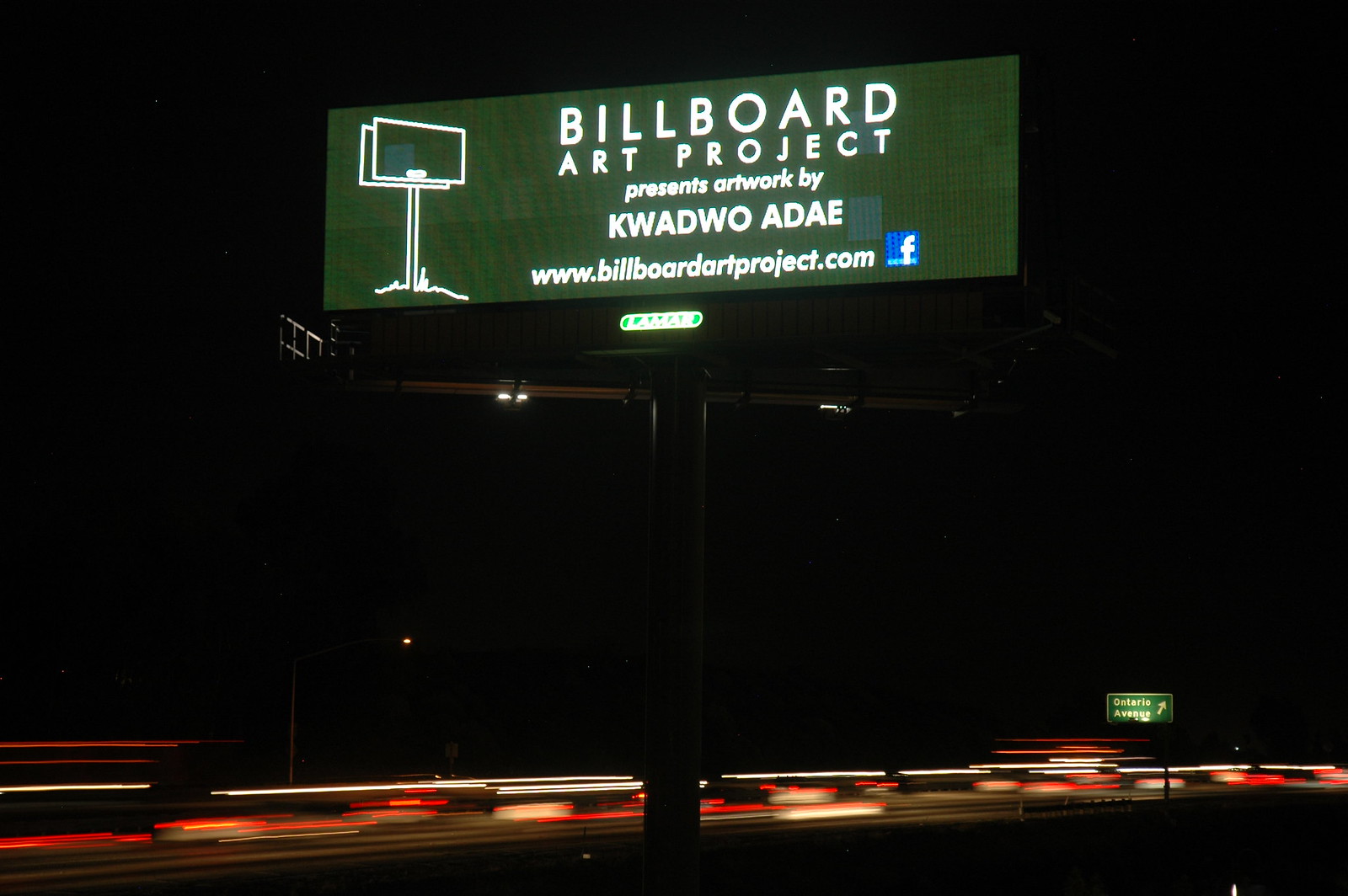The image captures a night scene under a black sky. The primary focus is a bustling highway where the blurred, red and white streaks of moving cars create a dynamic, speed-of-light effect across the road. In the bottom right corner, a road sign labeled "Ontario Avenue" with an arrow pointing up to the right is visible. Dominating the center of the image is a large green billboard. To the left, within the billboard, there is an inset photo of another billboard. The main text on the billboard reads: "Billboard Art Project presents artwork by Quad. Whoa a day" and includes a website: "www.billboardartproject.com." A Facebook logo appears below this text. At the base of the billboard structure, a lit-up sign reads "Lamar" in red and green colors, accompanied by illuminated white text below it. Despite the surrounding elements, the eye is naturally drawn to the prominent billboard at the forefront of this urban nightscape.